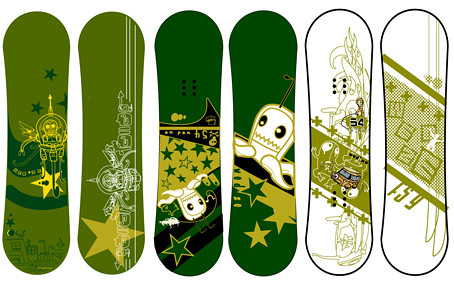This image features six snowboard or skateboard designs, arranged in a landscape orientation. Each board showcases a similar artistic style, likely indicating the same creator. The first two boards on the left are army green. The first one features a golden robot with a large golden star and dark green stars above its head, set against a cityscape at the bottom. The second board also has a big golden star, accompanied by a white sideways image. The next two boards are dark green, both depicting a golden octopus-like creature surrounded by golden and dark green stars, though the illustrations differ slightly. The last two boards are primarily white with army green sketches, which are more abstract and harder to discern. All six designs are artistic, potentially vectorized or created using Adobe Illustrator, and display varying shades of green, along with some text that's difficult to make out.